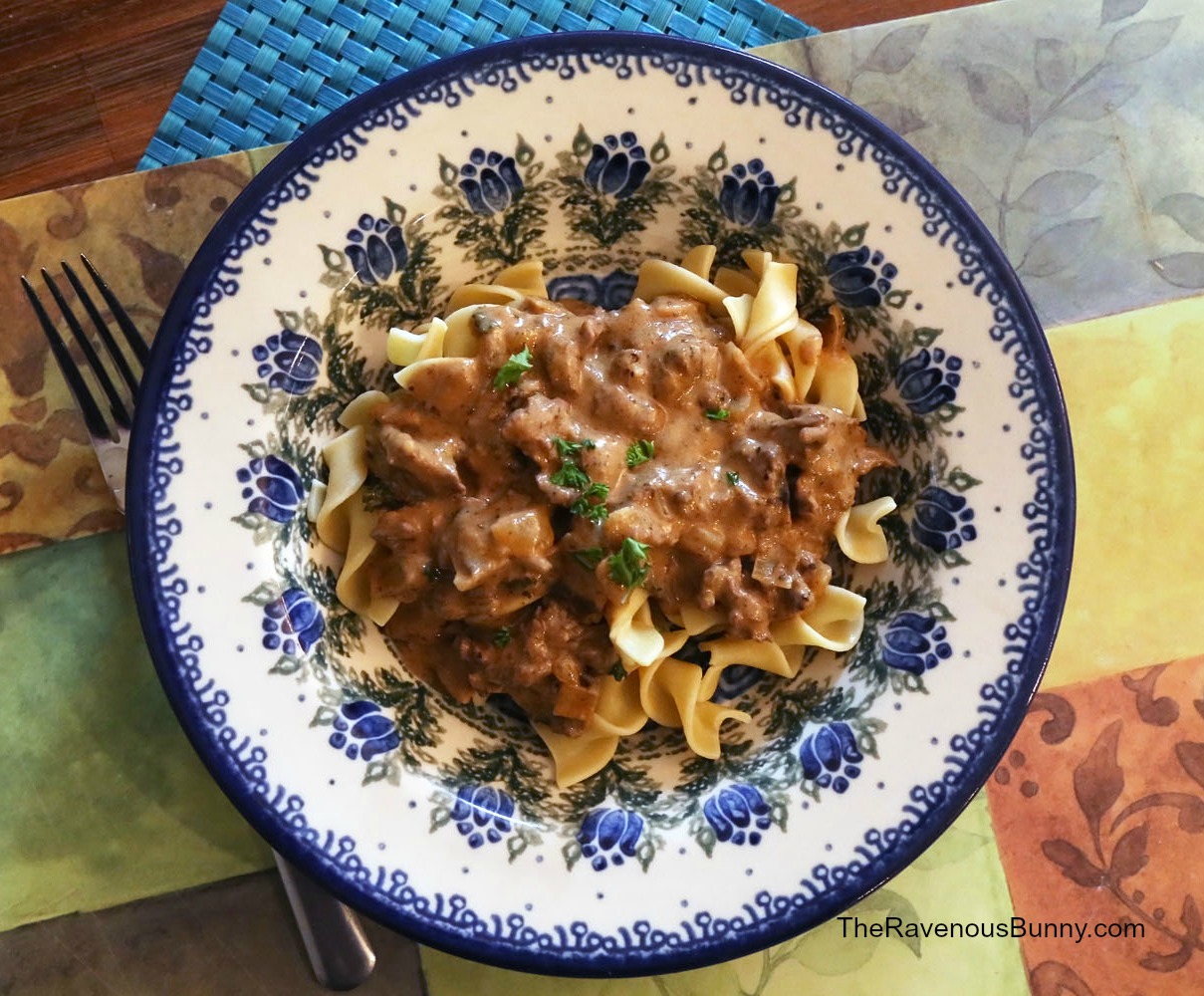The image features a close-up, overhead photograph of a delectable beef stroganoff pasta dish served in an intricately embroidered white bowl with dark blue patterns, which include floral and leaf motifs. The pasta, likely egg noodles, is topped with a rich, brown beef stroganoff sauce and garnished with either parsley or basil. The bowl sits on a vibrant checkered placemat displaying a mosaic of colors—yellow, blue, red, green—and adorned with leaf patterns. A fork is positioned to the left of the bowl, and a blue napkin or coaster peeks through at the top. In the bottom right corner of the image, the text "theravenousbunny.com" is printed.